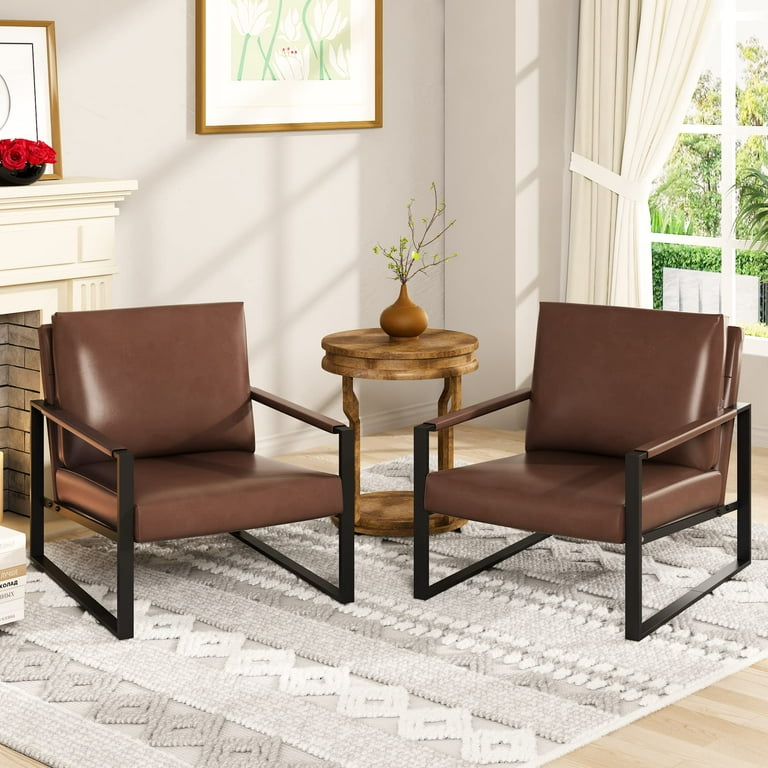In this cozy living room, the walls are painted a faint grayish hue, providing a serene backdrop. On the left side, a fireplace with a white mantle and hearth is adorned with wooden-framed pictures. The fireplace, featuring a mirror on the mantle along with a shallow vase of red roses, appears unused with clean bricks. Nearby, there are two low-set leather chairs, likely covered in a shiny tannish brown leather, with distinctive metal frames forming square-shaped arms and legs. These chairs are positioned diagonally facing each other atop a textured whitish-gray rug spread over the hardwood floor. Between the chairs is a round, two-layered oak coffee table with spindle legs, holding a wooden vase filled with branches and yellow flowers. To the right, just out of frame, a window with curtains pulled back lets in a shaft of sunlight, enhancing the room's warm ambiance.